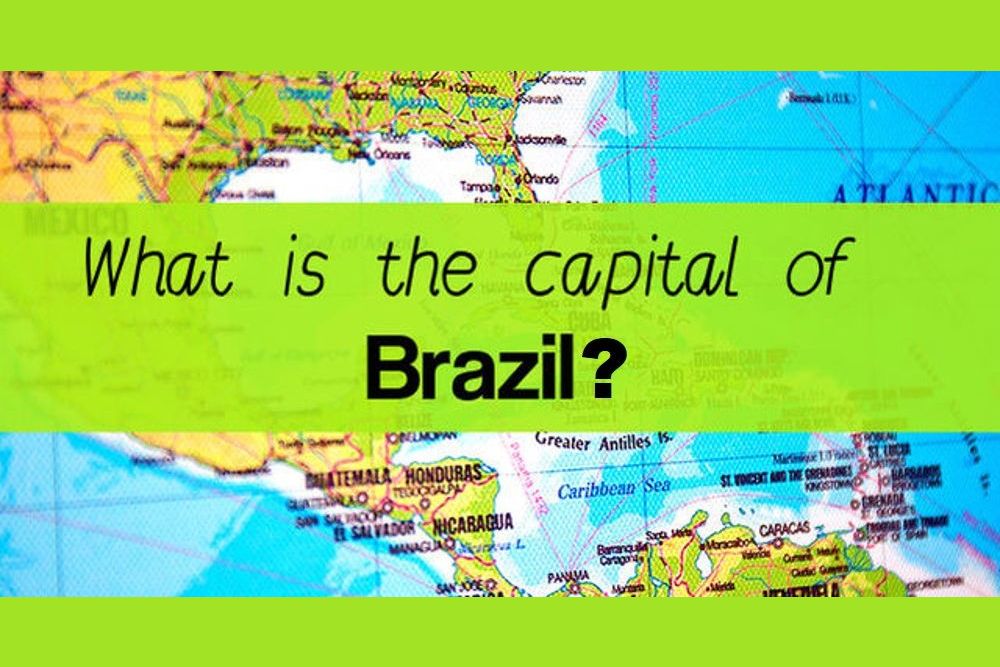The image is a rectangular map with a significant amount of detail and a central query. The top and bottom portions of the map are green, while a light green banner runs horizontally across the center. Written in bold black letters on this banner is the question, "What is the capital of Brazil?" with "Brazil" and the question mark in even bolder black text.

To the right of the map, the Atlantic Ocean is prominently featured in blue. On the top left corner, the map depicts parts of Texas, the Gulf of Mexico, and Florida. Below this area, Mexico and portions of Central America are visible, each labeled in black letters with names of places. Lines delineating states, territories, and countries crisscross the map.

The bottom right of the map shows the northernmost tip of South America, with location names in black writing that are too blurry to decipher clearly. Surrounding the continents, the water is white along the edges, blending into the blue of the ocean. The Atlantic Ocean is labeled in black letters, and a dark blue grid pattern spans the entire map, adding to the geographical details.